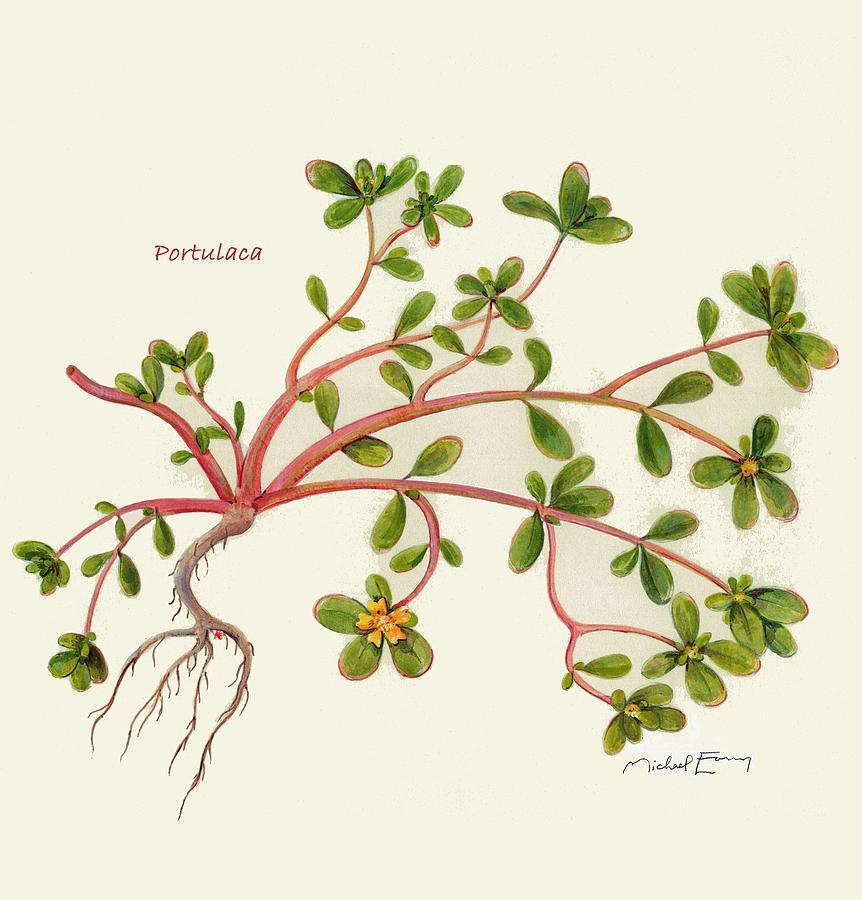This is a detailed and carefully rendered illustration of a plant set against an off-white, yellowish-beige background. The plant features reddish-pink stems and a visible brown root with smaller tendrils. Sprouting from the stems are several clusters of small, vibrant green leaves. Some of the clusters closer to the root display yellow flowers with five distinct petals. There are also rounded green leaves scattered throughout the plant. Notably, there is a maroon inscription on the left side that reads "Portulaca," indicating the plant species. The signature of the artist, Michael Avery, is present in the bottom right corner. This meticulous drawing captures the delicate structure and varied colors of the plant, showcasing elements like the reddish-pink stems, green leaves, yellow flowers, and the intricate root system.